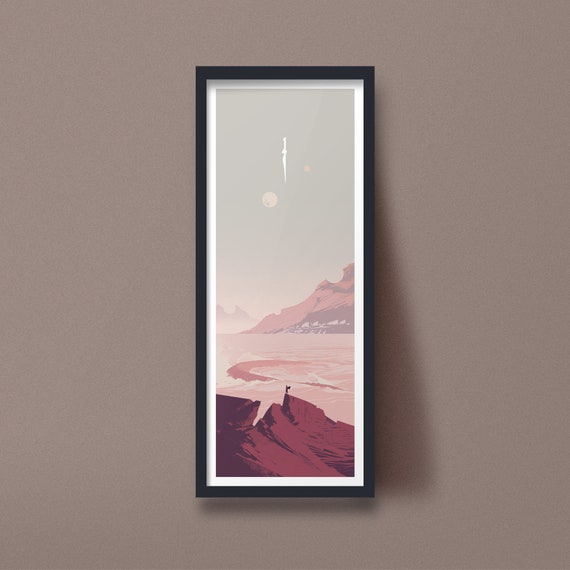The image showcases a long, vertically-oriented rectangular frame hanging on a taupe-colored wall. The frame is slender and black, enclosing a wide white mat. The painting within the frame depicts a desert landscape reminiscent of a canyon, characterized by jagged red peaks dominating the foreground. Beyond these peaks, the terrain extends into a broader desert area with another distinctive red mountain in the far background. The sky is painted in a very pale blue hue, complemented by the central presence of a white moon. There is also a subtle white streak across the grayish sky, adding a sense of depth to the scene. The color palette transitions from medium to darker pink tones, highlighting the silhouettes of the light mountains against the desolate landscape.